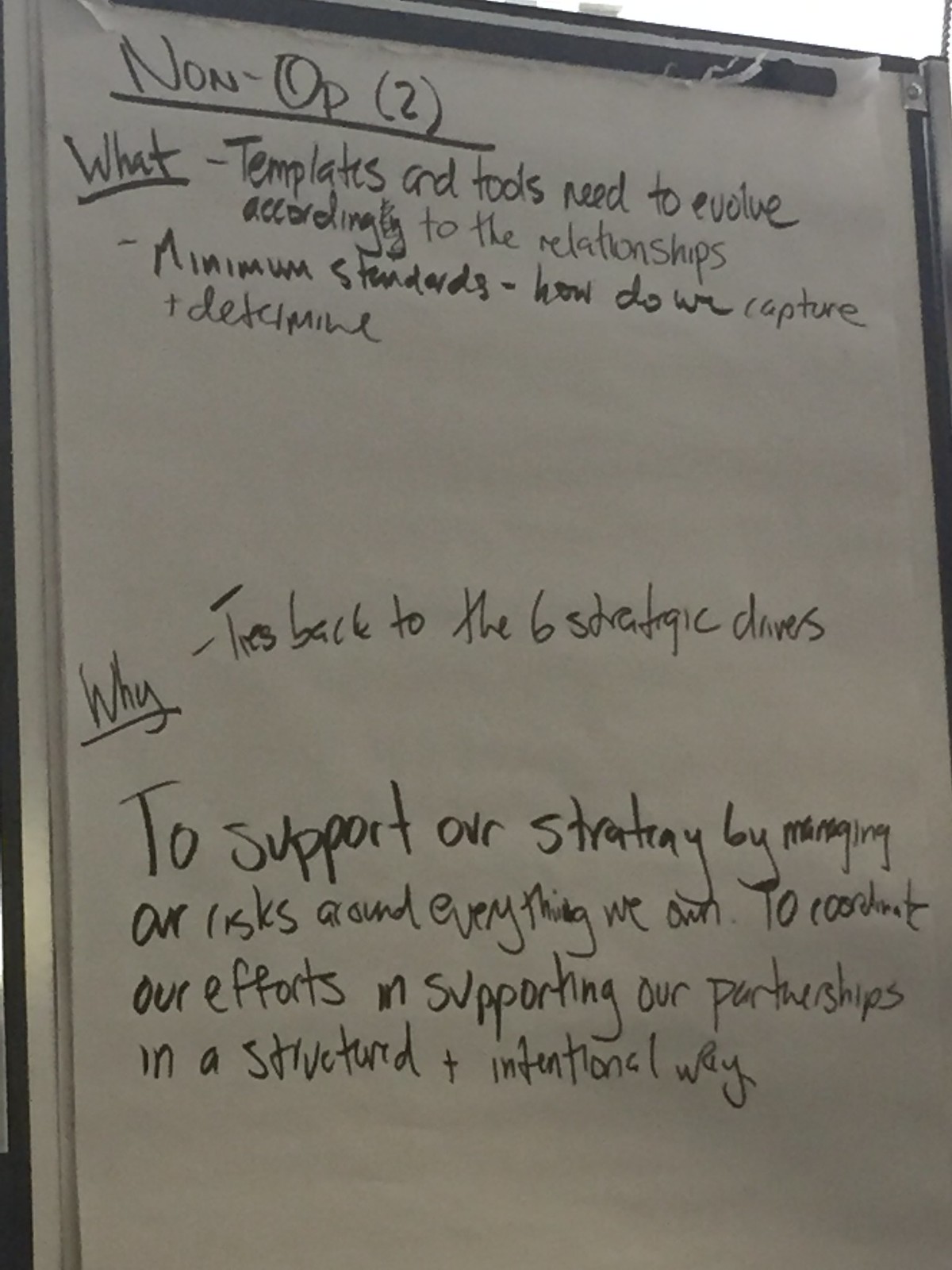A whiteboard-style piece of paper is displayed, its purpose centered around strategic management. The text, difficult to read due to poor lighting and inconsistent spacing, includes various templates and tools meant for evolving strategic parts. Key phrases emphasize avoiding pitfalls, disqualifications, and challenges, highlighted prominently in red. Amy Pecky is mentioned multiple times, possibly indicating her involvement or presence at the scene. The setting is unclear, adding to the overall ambiguous presentation of the strategic guidelines.